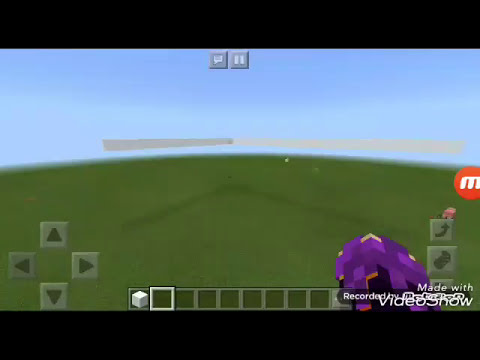This is a screenshot from a live-stream of a Minecraft-like video game, possibly filmed on a laptop screen. The image shows a barren grassland with nothing built, under a clear blue sky. There’s a long, gray, and tan bar on the horizon casting a shadow on the grass. The game interface includes directional arrow keys (up, down, left, right) in the bottom left corner and an inventory at the bottom center, with the first slot containing a white block and the second slot highlighted but empty. At the top center of the screen, there are pause and chat buttons. The bottom right corner features a purple blob, potentially a controller, along with the "video show" program label in white font. A small "M" icon is also visible on the bottom right, and what looks like a player's hand with a purple wrist is faintly captured in the shot.